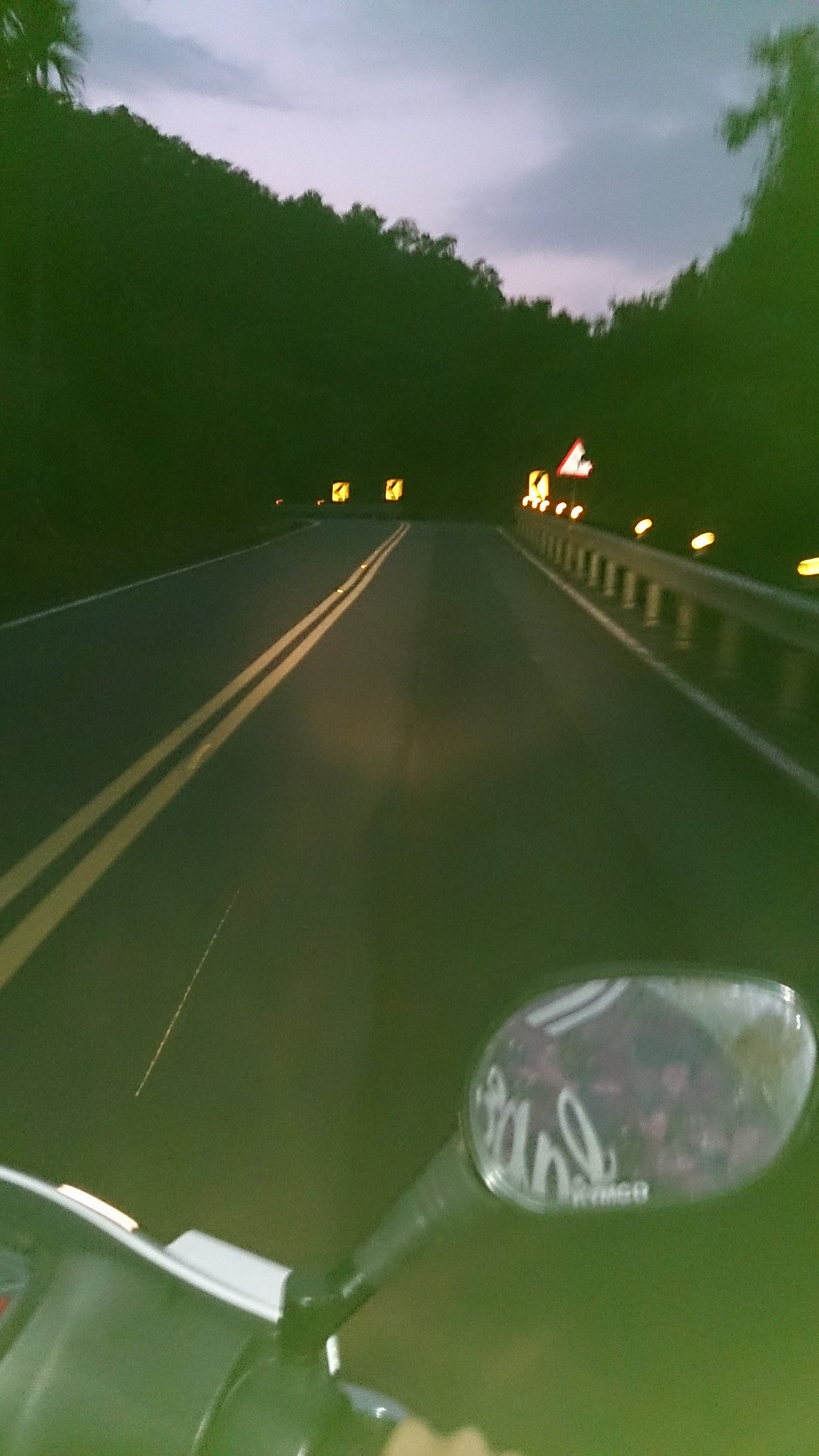A lush forest surrounds the scene, with a dense canopy of vibrant green leaves overhead and a variety of leafy underbrush covering the ground. Stretching ahead is a narrow asphalt road, clearly divided by a central line. In the distance, there are several yellow road signs with arrows curving to the left, indicating a winding route ahead. A prominent white triangle sign with a red border also catches the eye. The photograph is taken from a motorcycle, evident from the right-side mirror which reflects part of the rider's helmet, featuring cursive text, possibly "Romeo." The helmet is primarily white accented with a black stripe. The motorcycle's handlebar is partially visible, along with a section of its white trim, adding to the dynamic composition of the image.